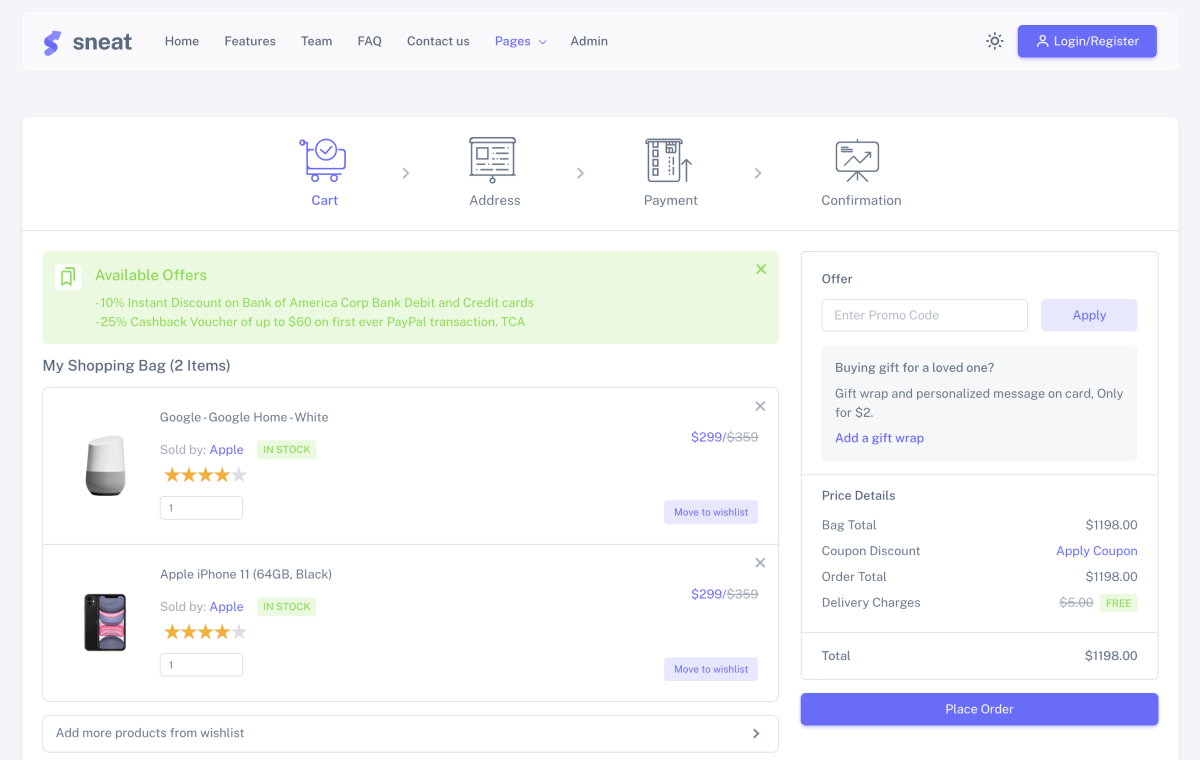Screenshot Description:

The screenshot displays a website with a white background. At the top, the site title "SNEET" appears in bold black lettering. Below the title, there is a horizontal menu bar featuring several options in blue text: "Home," "Features," "Team," "FAQ," "Contact Us," and more. To the right of this menu, options such as "Admin" and icons for "Login/Register," "Profile," and "Cart" are visible.

Beneath the main menu, there is a section highlighting available offers, enclosed in a green rectangle. The offers include:
- A 10% instant discount on Bank of America Corp bank debit and credit cards.
- A 25% cashback voucher, up to $60, on a first-ever PayPal transaction.

Following the offers section is the user's shopping cart overview, titled "My Shopping Bag" with a note indicating two items. The items listed are:
1. Google Home (White), sold by Apple, in stock, rated four stars, priced at $299, with an option to "Move to Wish List."
2. Apple iPhone 11 (64 GB, Black), sold by Apple, in stock, rated four stars, also priced at $299, with similar options for wish list management.

An additional feature allows users to "Add More Products from Wish List." There's a section for applying an offer, indicated by a box and a blue "Apply" button. 

At the bottom of the screenshot, an invitation to purchase a gift for a loved one is highlighted within a blue rectangle, prompting the question, "Buying a gift for a loved one?"